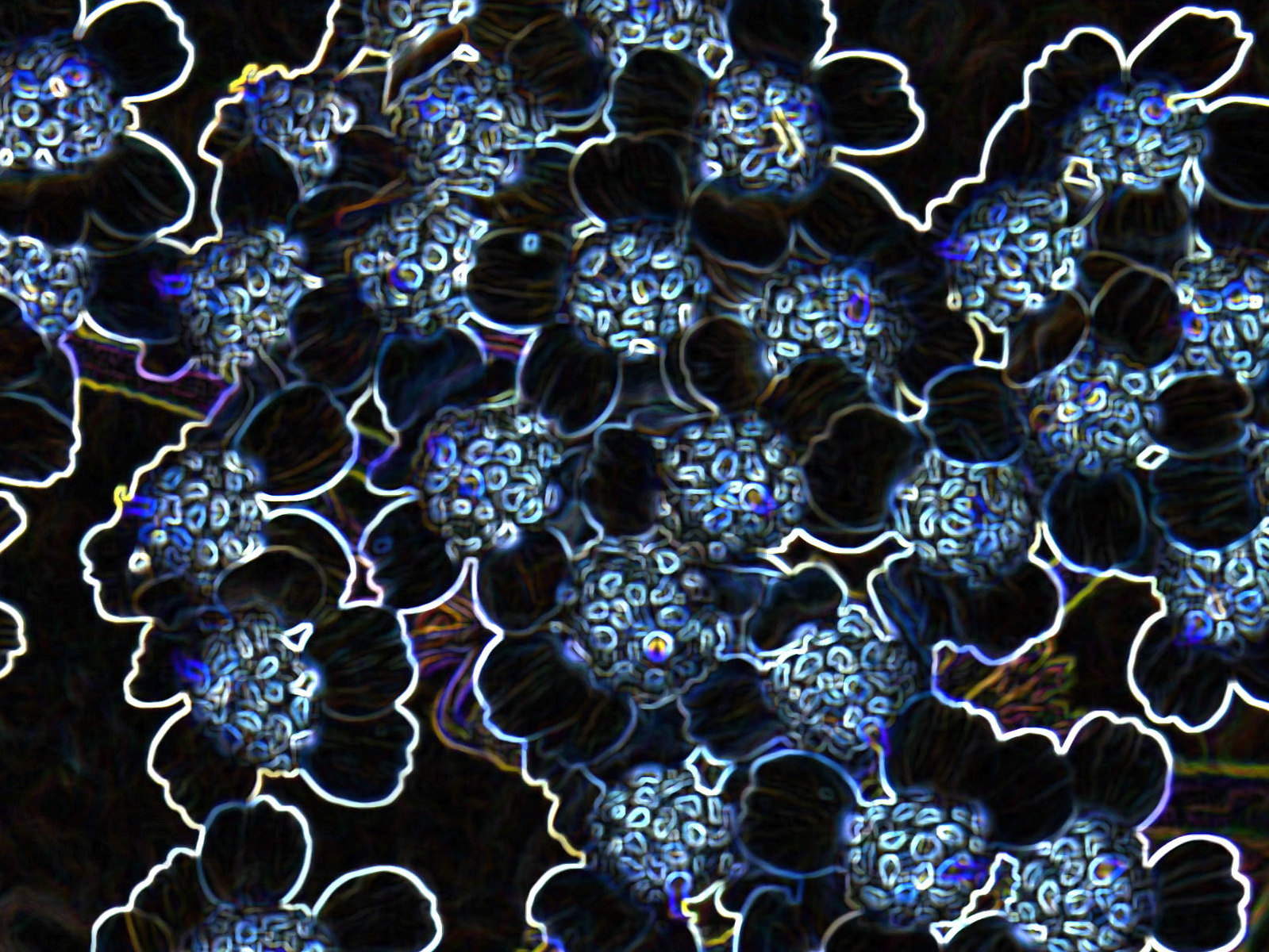The image features a mesmerizing black background adorned with intricate, bright neon colors, predominantly shades of blue including light blue, dark blue, navy blue, sea blue, and sky blue. These vibrant blues form circular clusters, giving the impression of floral patterns, reminiscent of hydrangea heads. Interspersed among the blue are white lines and squiggles that add to the complexity of the design, some of which have touches of yellow and purple, enhancing the visual appeal. The overall effect is akin to a dazzling black light display, with the neon hues glowing brilliantly against the dark backdrop. The arrangement and the vivid colors might evoke thoughts of an elegant wallpaper design or a modern abstract artwork created digitally.